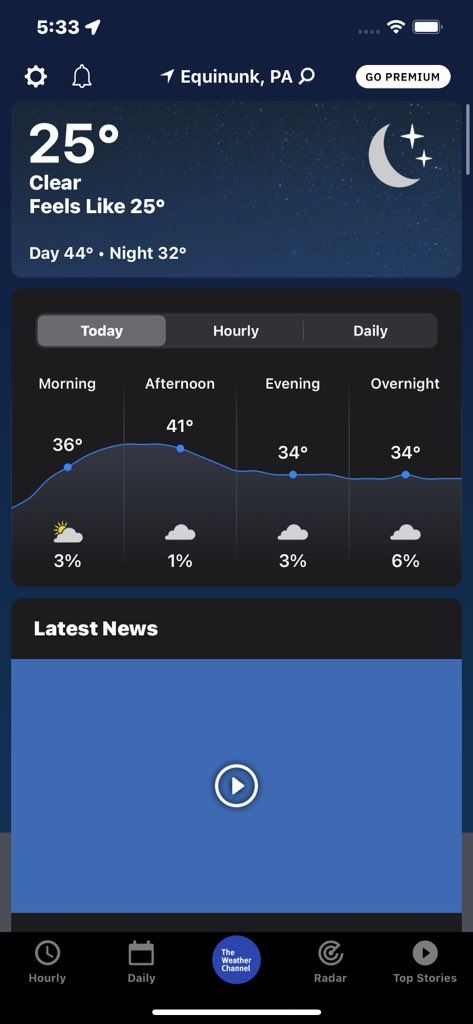A detailed nighttime screenshot from a smartphone showing a weather update for Equinunk, Pennsylvania at 5:33 AM. The phone displays full Wi-Fi connectivity and a fully charged battery but no cellular service. The weather app, likely from The Weather Channel, indicates it's a clear night with a temperature of 25°F, which feels like 25°F. The forecast predicts a high of 44°F during the day and a low of 32°F at night. Additional hourly forecasts indicate temperatures of 36°F in the morning, 41°F in the afternoon, and 34°F both in the evening and overnight. A white banner at the top offers a premium upgrade. Below the weather details, a video section titled "Latest News" is ready to play. The app features a blue Weather Channel logo and navigational tabs at the bottom for 'Hourly,' 'Daily,' 'Radar,' and 'Top Stories.' Moon and stars icons signify nighttime.